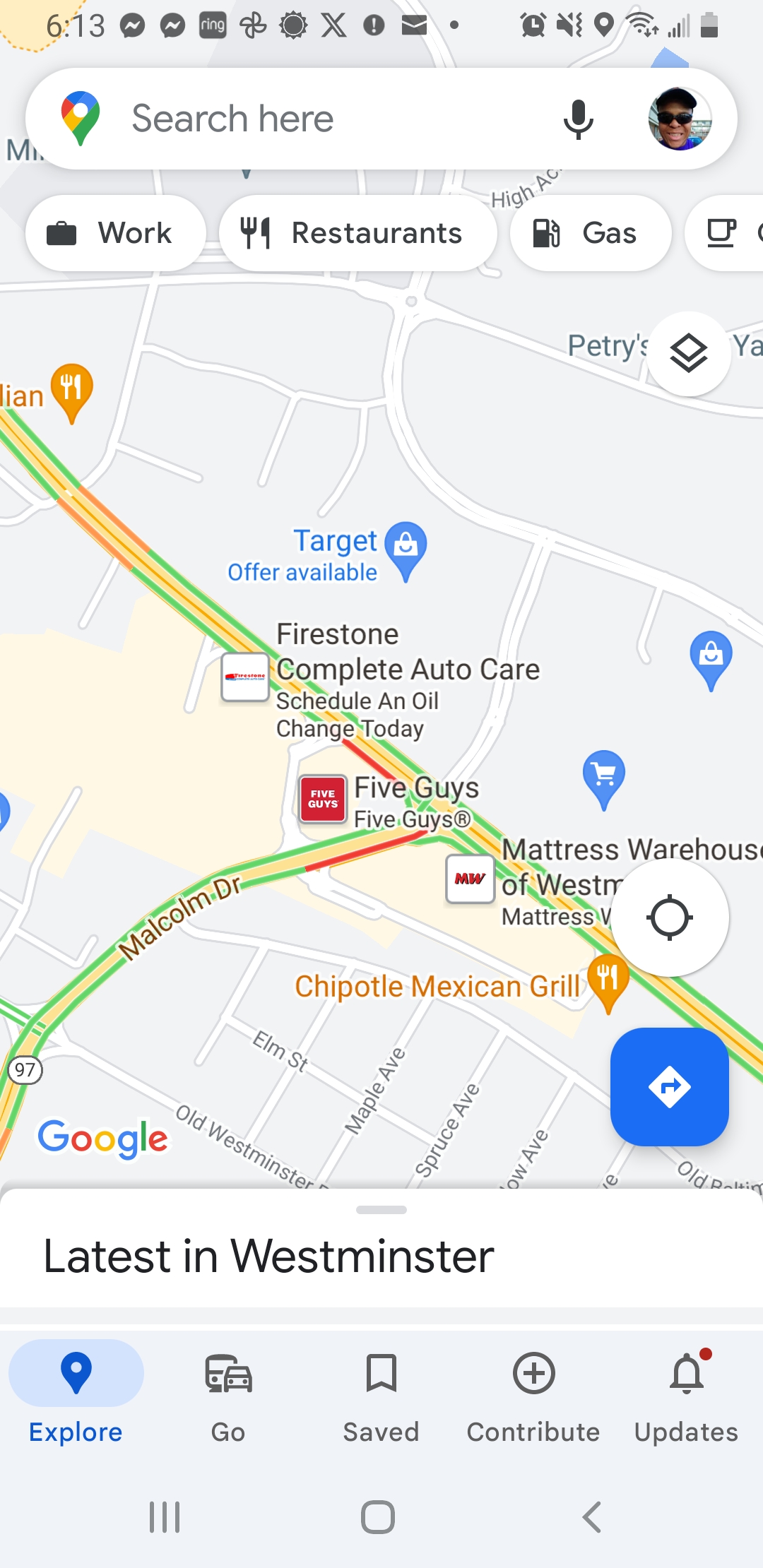A screenshot of a smartphone's display showing the time as 6:13 AM/PM. The status bar at the top of the screen includes various icons, such as a medium-charged battery indicator. The main section of the screen displays the Google Maps app, with a prominent search bar that reads "Search here." To the right of the search bar, there is an icon for voice commands and a small circular profile picture featuring a dark-skinned man wearing a black cap, black sunglasses, and a blue shirt.

Below the search bar, several quick-access buttons are visible, labeled for categories like "Work," "Restaurants," and "Gas." The map itself highlights the area around two intersecting streets: Malcolm Drive and a second, unnamed street. Landmark icons for Target, Firestone Complete Auto Care, and Chipotle Mexican Grill are also shown on the map. Finally, the bottom left corner displays the Google logo, signifying the app's developer.